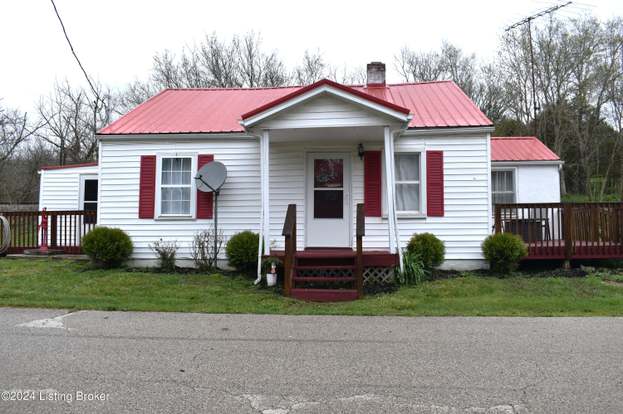The photograph depicts a modest, small white house with red shutters on two front windows, a white storm door, and a distinctive reddish-tiled roof. The house exudes a farmhouse-like charm and is surrounded by early spring greenery, including green grass and shrubs. A prominent satellite dish on a pole, a large TV antenna, and a small chimney are visible on the roof. There are two additions attached to the house: one on the right, featuring a redwood porch with slats and possibly a black grill, and another on the left which resembles a white-sided shed with a similar roof. In the background, bare trees are interspersed with budding leaves, indicative of the early spring season. The house is fronted by a paved road, which appears slightly wet as if it has recently rained. The image is slightly longer than it is tall, and in the bottom left corner, white lettering reads, "2004 Listing Broker," suggesting that the house is probably for sale. The overall setting is bright and clear with natural lighting, and the sky is somewhat cloudy.